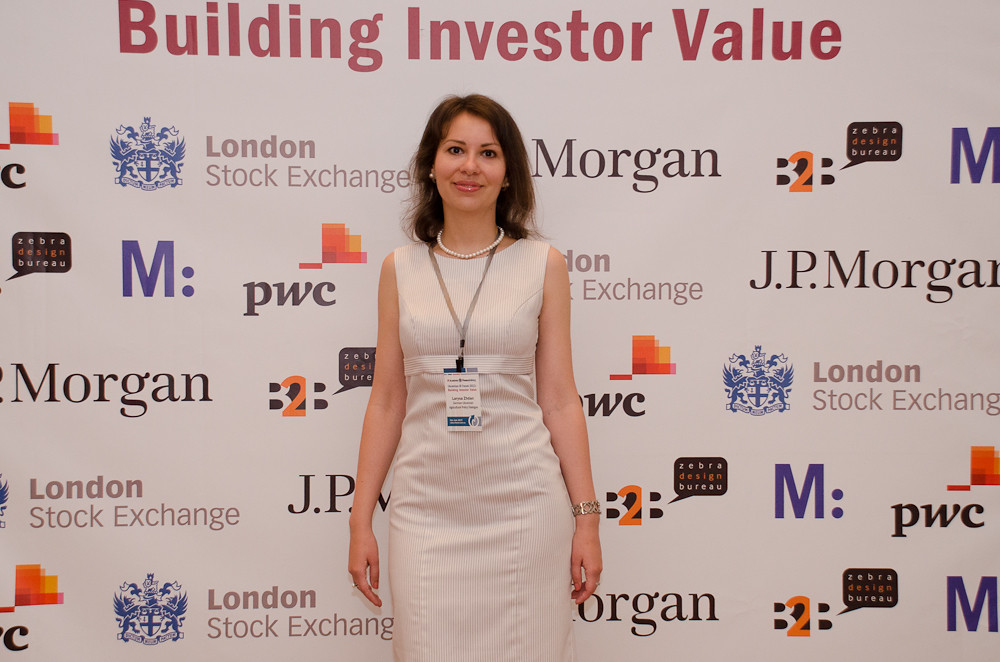In the image, a woman stands upright in front of a corporate advertisement backdrop, likely at a conference or convention. Dressed in an off-white dress with a faint vertical line pattern, she is accessorized with a pearl necklace and earrings, and a silver wristwatch on her left wrist. Her brown hair frames her face as she stares directly into the camera with a subtle smile. Around her neck hangs a lanyard with a blue and white pass, held by a black rope, which reaches the middle of her chest. The backdrop features a white wall with red text reading "Building Investor Value," and logos of several organizations such as the London Stock Exchange (with a blue heraldic emblem), J.P. Morgan, and PwC, arranged in five repeating rows. The setting appears to be at a corporate seminar or meeting, and she poses confidently in front of the sponsors' logos.